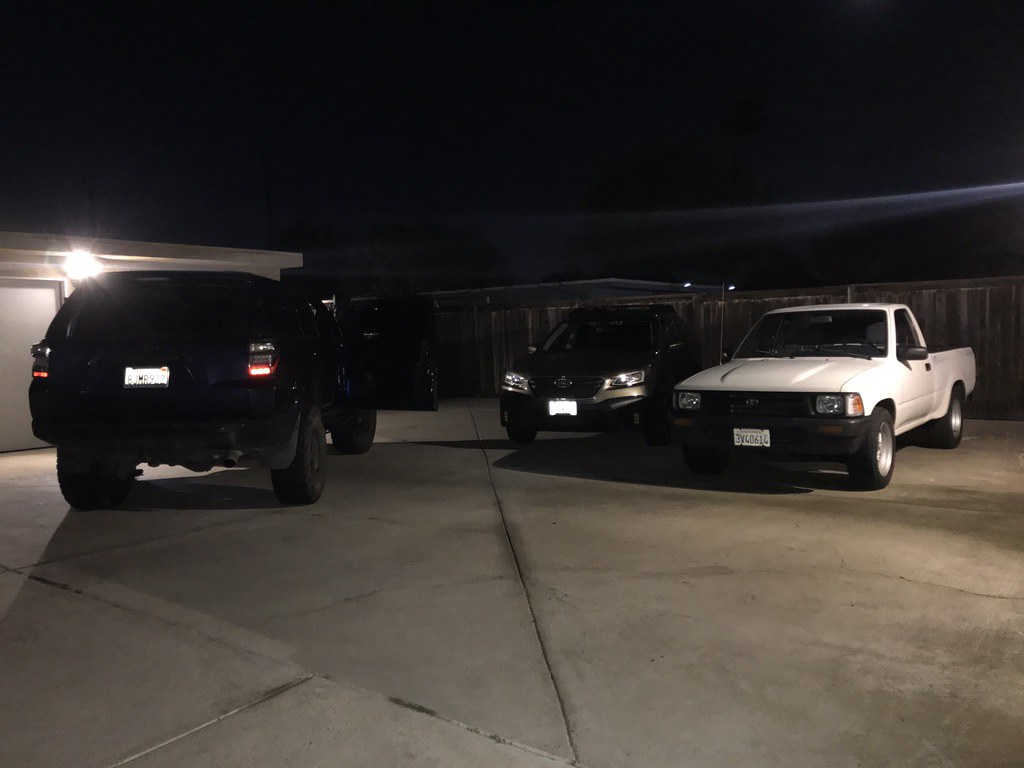This nighttime photograph depicts a large, slightly cracked concrete driveway bordered by an old brown wooden fence. The sky is pitch black, and the faint silhouette of trees is visible in the background. On the left side of the image stands a light-colored house with part of its white garage door and roof showing. Three vehicles are parked in the driveway: an older white Toyota pickup truck facing the camera, a dark-colored Subaru Outback positioned next to the Toyota and also facing the camera, and a navy blue Toyota 4Runner with its driver's side door open, facing away from the camera. Behind the vehicles, the closed double garage door is visible, illuminated by a light situated between the doors. The setting suggests a gathering, although no people are present in the photo.